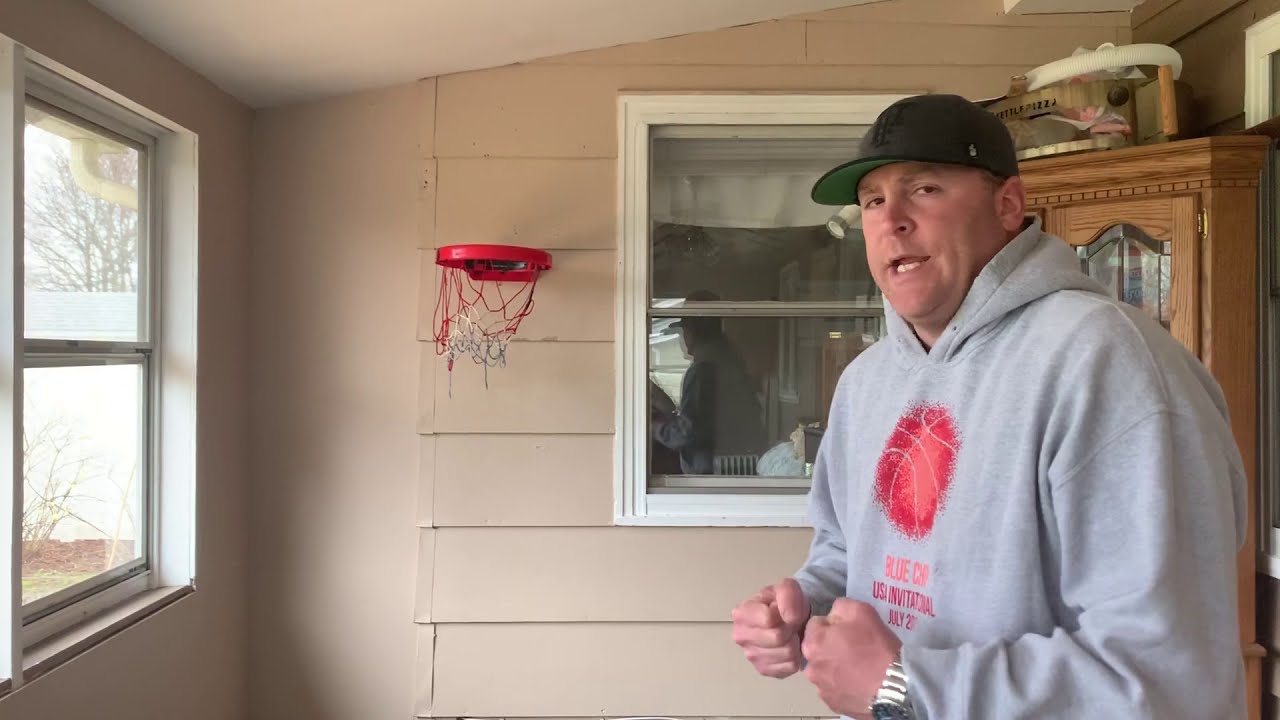In a cozy, light-tan room adorned with wood slats, a mid-40s Caucasian man stands poised, flexing his arms with his hands clenched into fists. He is captured looking directly at the camera, his mouth slightly open, revealing his lower teeth as if speaking. Wearing a black baseball cap with a green underside and a gray long-sleeve hoodie featuring a basketball graphic and the text "Blue Cap U.S. Invitational July," he exudes casual confidence. A silver watch adorns his left wrist. The room, reminiscent of a patio or mudroom, contains an assortment of items: a window with a white frame, an indoor child’s plastic basketball hoop, a brown oak chest, and hints of a curio cabinet. The ambiance is both homely and bustling, with objects indicative of an active household.